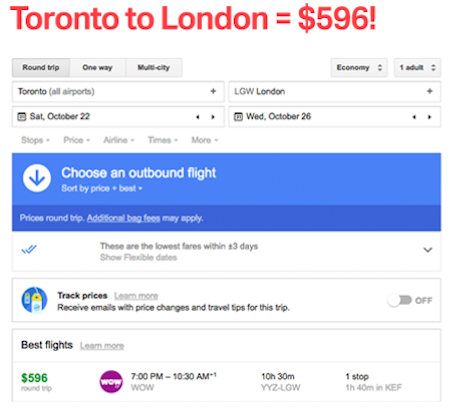Screenshot of a travel booking website featuring a predominantly white background with a central blue bar. At the top, a red headline announces: "Toronto to London = $596!" Just below, navigation options include tabs for "Round Trip," "One Way," and "Multi-City." On the right side, dropdown menus are available for selecting the travel class ("Economy") and the number of travelers ("One Adult").

Beneath the navigation options, the departure city is displayed as "Toronto" with a departure date of "Saturday, October 22nd." Adjacent to it, the destination is shown as "LGW London" with a return date of "Wednesday, October 26th." 

Below these details, five pale grey filter tabs are provided, labeled "Stops," "Price," "Airlines," "Times," and "More." Directly underneath is a light blue block with a white circle and a downward arrow, which includes the text: "Choose an outbound flight, sort by price or best." This is followed by a dark blue block containing the information: "Prices, round trip, additional bag fees may apply."

Further down, a white block with two blue arrows highlights the message: "These are the lowest fares within three days. Show flexible dates." Finally, there are options for "Track prices," currently set to "Off," and "Best flights" showing a fare of $596 for a flight departing at 7:00 p.m. and arriving at 10:30 a.m. with WOW Airlines, noting that the flight includes one stop.